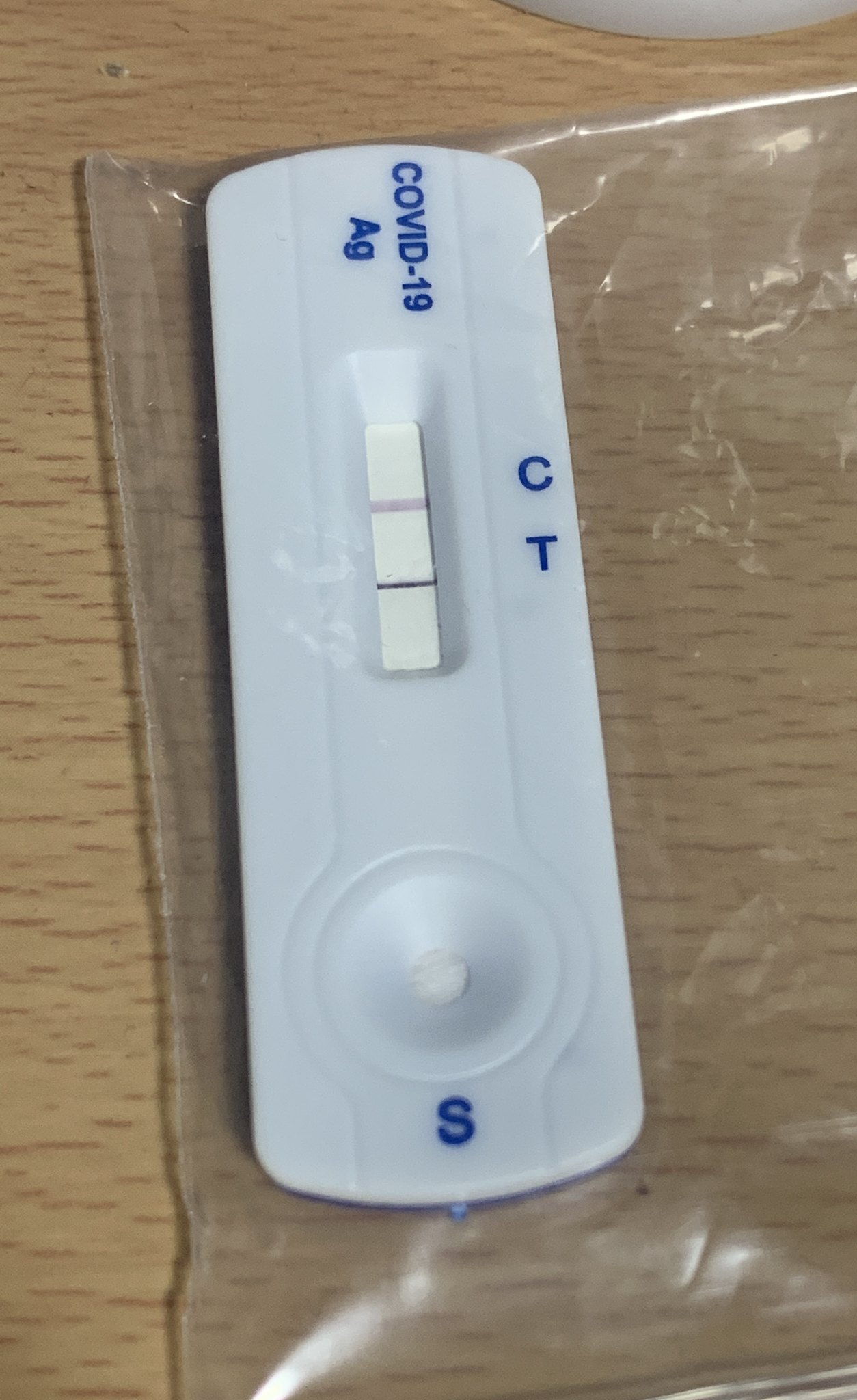A highly detailed close-up image reveals a COVID-19 test, which is prominently positioned as the focal point of the photograph. The test is encased in a transparent plastic bag, lying on a table with a light brown surface accentuated by darker brown streaks. At the very top of the image, a sliver of white is visible, though indistinguishable.

Despite the clear plastic bag’s transparency, one can discern that the test has settled at the bottom. A subtle reflection of light emanates from the lower edge of the bag. The test itself is rectangular with gently curved top edges and features several blue inscriptions. "COVID-19 AG" is prominently labeled in blue, while the right side bears the notations "C" and "T" in the same blue hue. Additionally, at the bottom, the letter "S" is also marked in blue.

The testing area shows two distinct lines within the white testing window, suggesting a positive result, with one line darker than the other. There is also a circular section and a designated area for sample application, completing the meticulous details of this essential diagnostic tool.